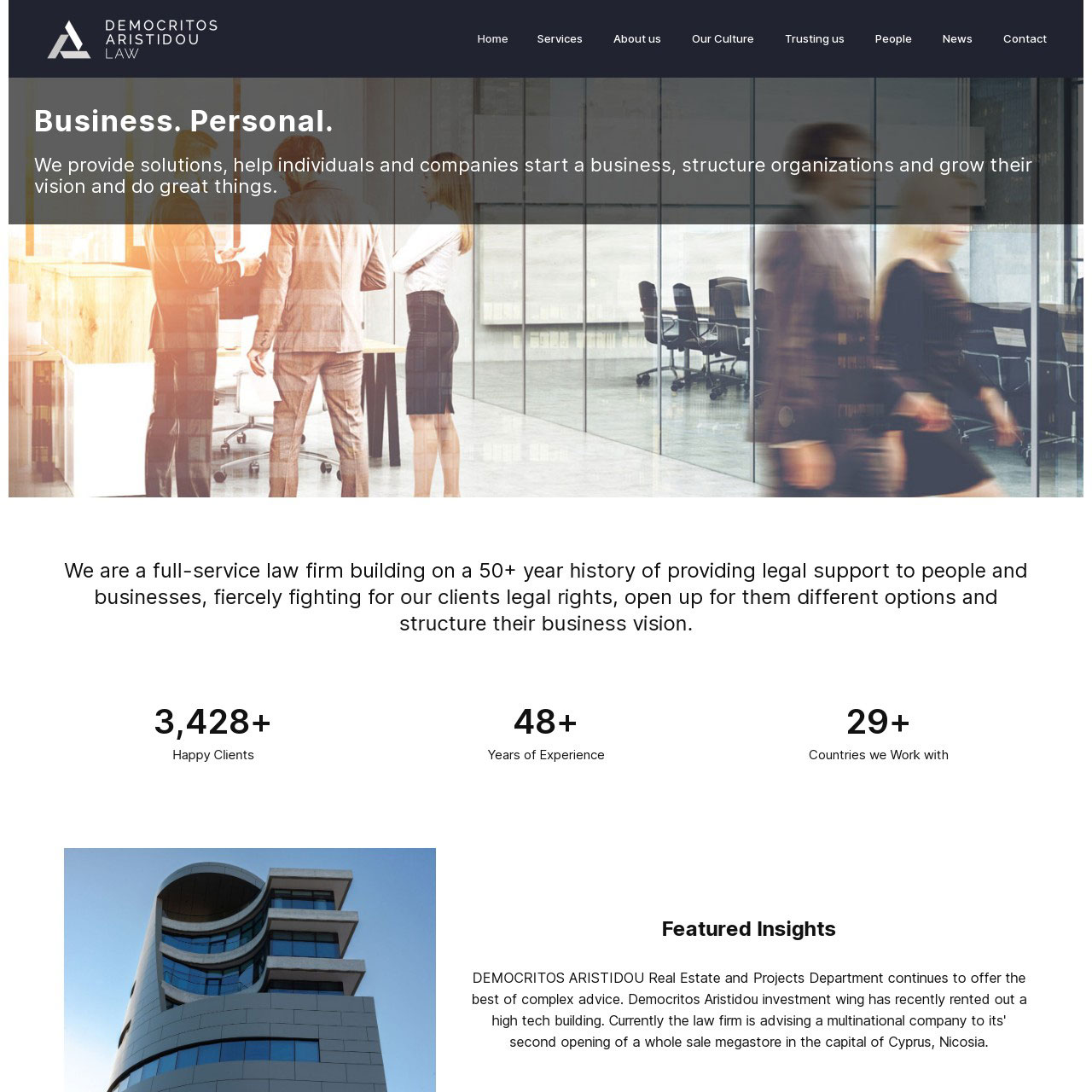**Caption:**

The image showcases the homepage of the law firm's website, "Demo Crittles Artist Edo Law." At the top of the page, the tagline "Business, Personal" reflects the comprehensive nature of their services. Below this, a statement highlights the firm's mission: "We provide solutions, help individuals and companies start a business, structure organizations, and grow their vision to achieve great things."

Centrally positioned on the homepage, the text emphasizes the firm's extensive experience with the proclamation, "We are a full-service law firm building on a 50+ year history of providing legal support to people and businesses." It underscores their commitment to advocating for clients by stating, "We fiercely fight for our clients' legal rights, open up various options, and structure their business vision."

Further down the page, impressive statistics boast the firm’s global reach and client satisfaction: "34,000+ happy clients in 29 countries."